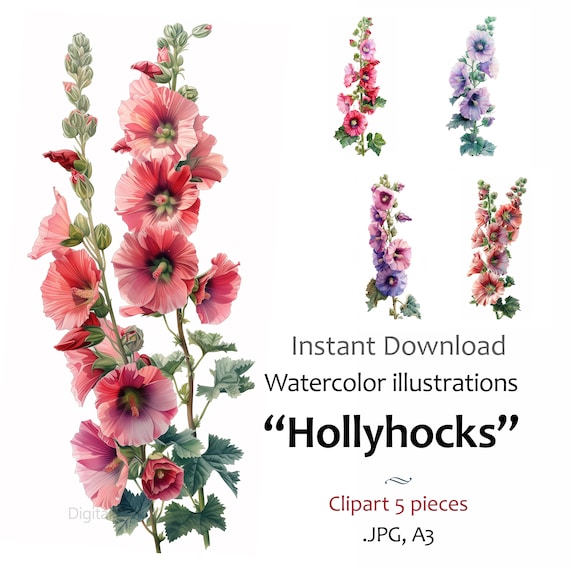This image showcases detailed watercolor illustrations of hollyhocks against a white background. On the left-hand side, two tall stems with green, spade-shaped, jagged leaves display pink and red flowy flowers, some of which are still buds. These stems extend vertically from the bottom to the top of the image. In the upper right-hand corner, there are four additional hollyhock illustrations, each featuring single stems with various flower colors: pink and red, violet, pink and violet, and red and white. All these flowers exhibit similar spiky leaves, and unopened green buds among the blooms. Beneath these illustrations, black text reads "Instant Download, Watercolor Illustrations, Hollyhocks," followed by "Clipart Five Pieces, JPEG, A3."